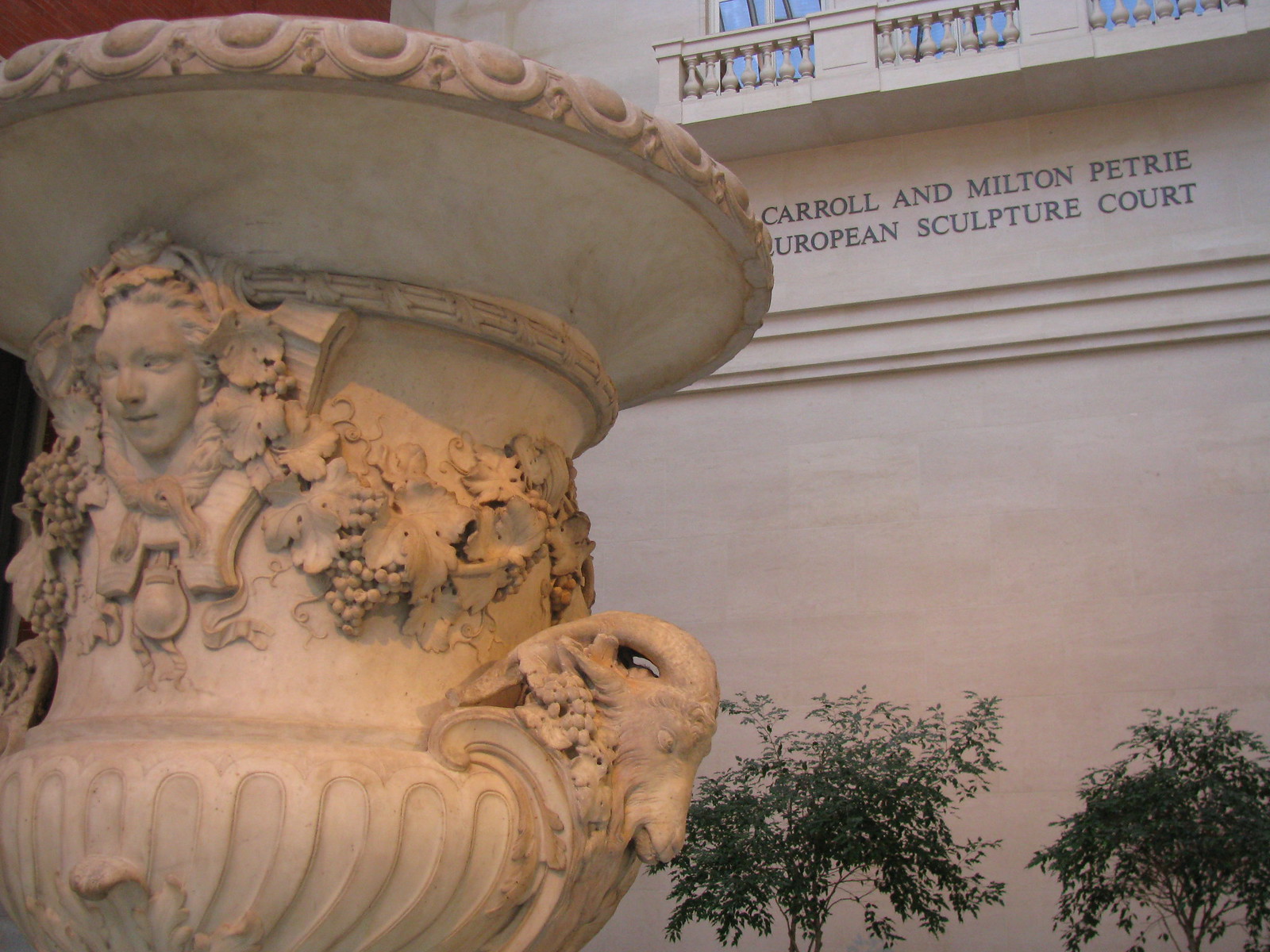In this photograph, a decorative white stone urn stands prominently in the foreground of a large, stone-block building identified by the black text "Carol and Milton Petrie European Sculpture Court." The urn, taking up nearly half of the image, is intricately adorned with a goat's head on one side and a human face on the front, accented by clusters of grapes and leaves cascading down its sides. The building itself features multiple double-paned windows and a small stone balcony with a matching stone railing at the top. To the bottom right of the image, small green-leaved trees peek into the frame, adding a touch of nature to the scene. The overall setting suggests an outdoor courtyard, possibly part of a museum dedicated to European sculptures.